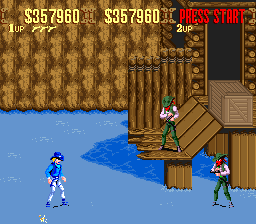In this vibrant, cartoon-styled screenshot from a video game, we see a character dressed in a baseball catcher's gear, though he isn't on a baseball field. The character is clad in a backward cap, a long-sleeved blue shirt, fitted white pants, and blue shoes. Opposing him are two distinct figures garbed in long-sleeved, pinkish shirts and fitted green stretchy pants. One of these figures sports an unmistakably alien face, while the other's face is somewhat concealed, lacking clear detail and definition. The setting features a richly textured brown and gold wall, adorned at the top with the prominently displayed amount of $357,960 written twice, flanking the center, with "Press Start" appearing to the right.